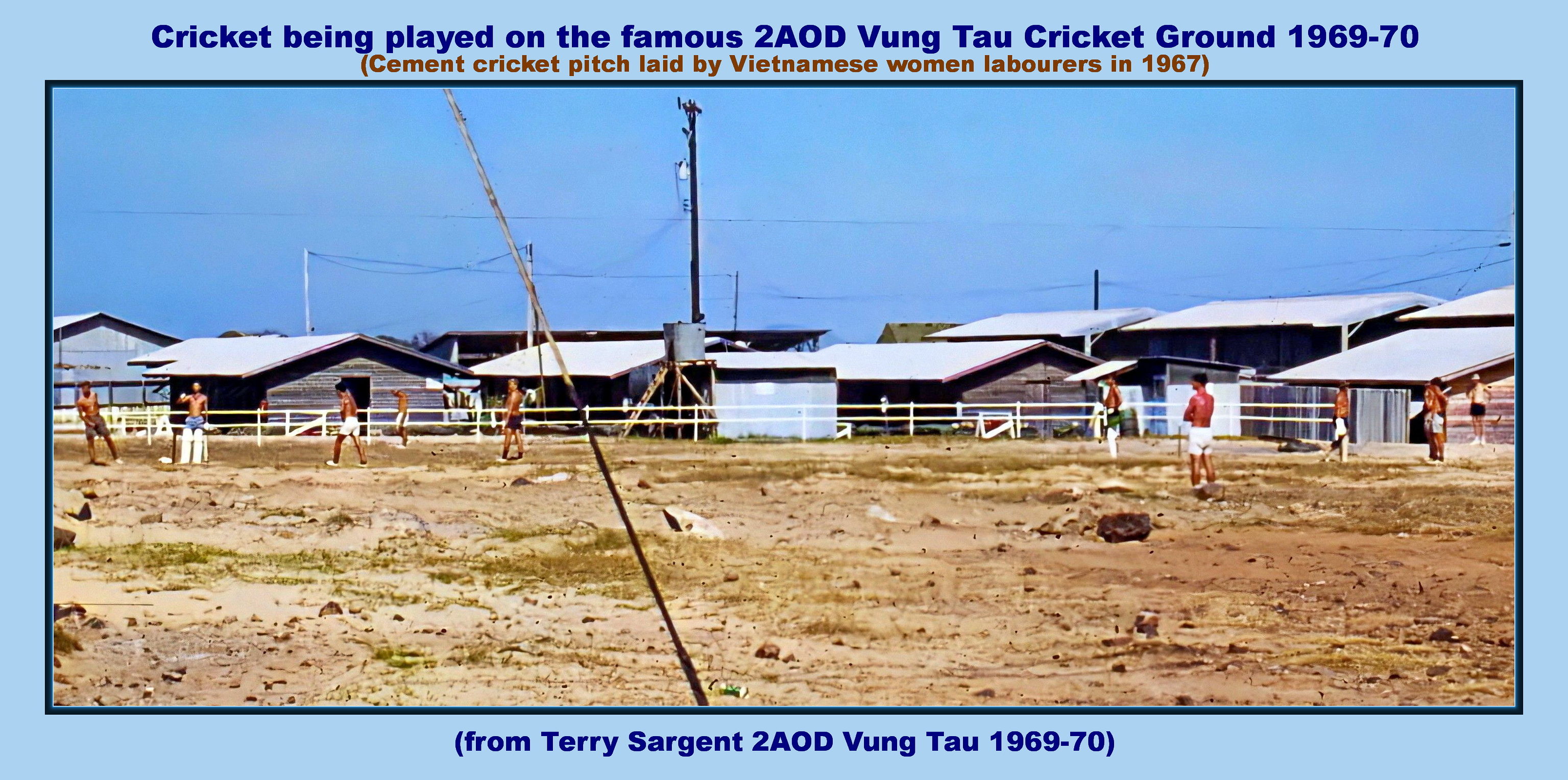The vintage photograph captures a moment from 1969-1970 at the famous 2AOD Vung Tau Cricket Ground during the Vietnam War. The image features shirtless young men, likely soldiers, enjoying a game of cricket on a rocky, uneven field dotted with dry vegetation and dirt patches. One player, wearing pads and gloves, is poised with a bat, while others are scattered across the field, suggesting active play. The sky is clear and blue, enhancing the sense of a hot day. In the background, multiple small buildings with tin roofs, identified as barracks, along with white fencing, telephone poles, and electrical wires, are visible. The photograph is bordered in blue with captions in dark blue and brown fonts, noting, "Cricket being played on the famous 2AOD Vung Tau Cricket Ground 1969-1970" and "Cement cricket pitch laid by Vietnamese women laborers in 1967." The footnote attributes the photo to Terry Sargent, 2AOD, Vung Tau 1969-1970, emphasizing its historical context.